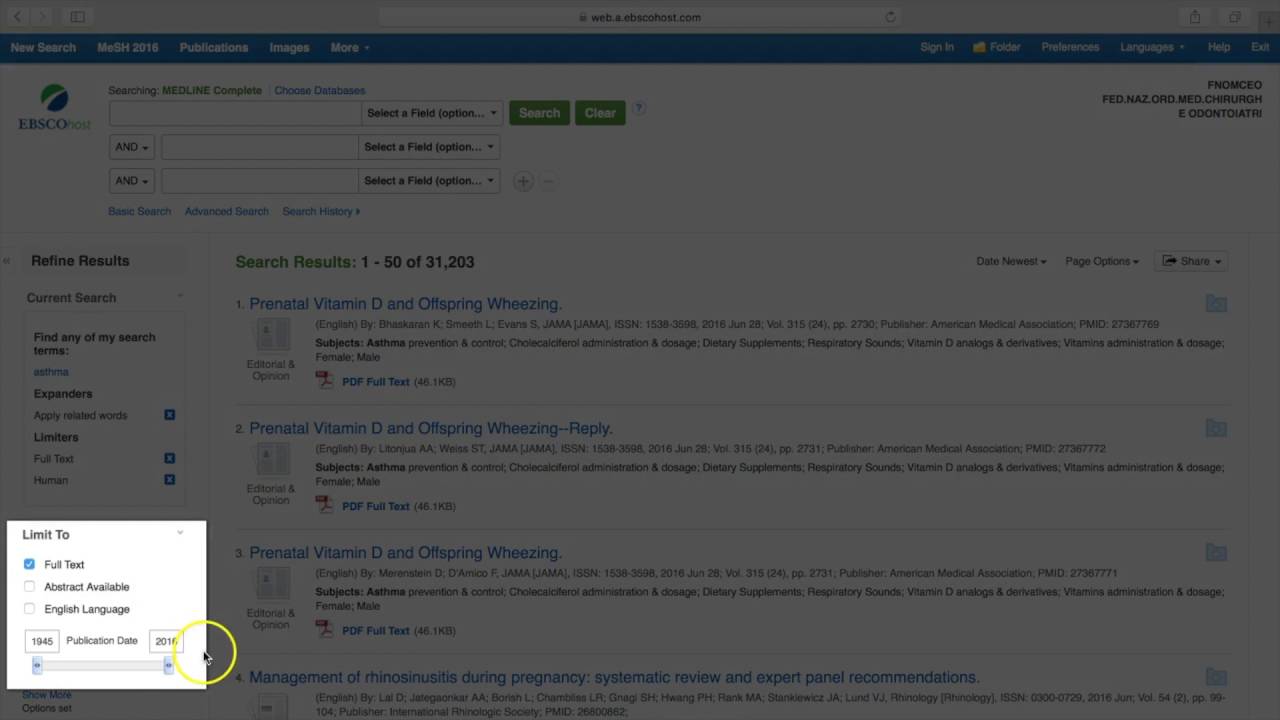This is a detailed screenshot of a product website, primarily tinted in black to focus attention on a pop-up window located at the bottom left. The underlying website features a prominent blue navigation bar across the top, which hosts several white buttons: "News," "Search," "MESH 2016 Publications," and "Images and More" (the latter being a drop-down menu).

On the right side of this blue bar are additional white links: "Sign In," "Folder," "Preferences," "Languages" (another drop-down menu), "Help," and "Exit." Below this, the interface includes three vertically-stacked input fields. The top field appears to be a search bar, accompanied by green "Search" and "Clear" buttons to its right. Adjacent to each of these fields is a drop-down button labeled "Select a Field."

The highlighted pop-up in the bottom left is focused on advanced search options, labeled "Limit to." This section presents three checkboxes for filtering search results by "Full Text," "Abstract Available," and "English Language." Additionally, there is a publication date range slider for further refining search criteria.